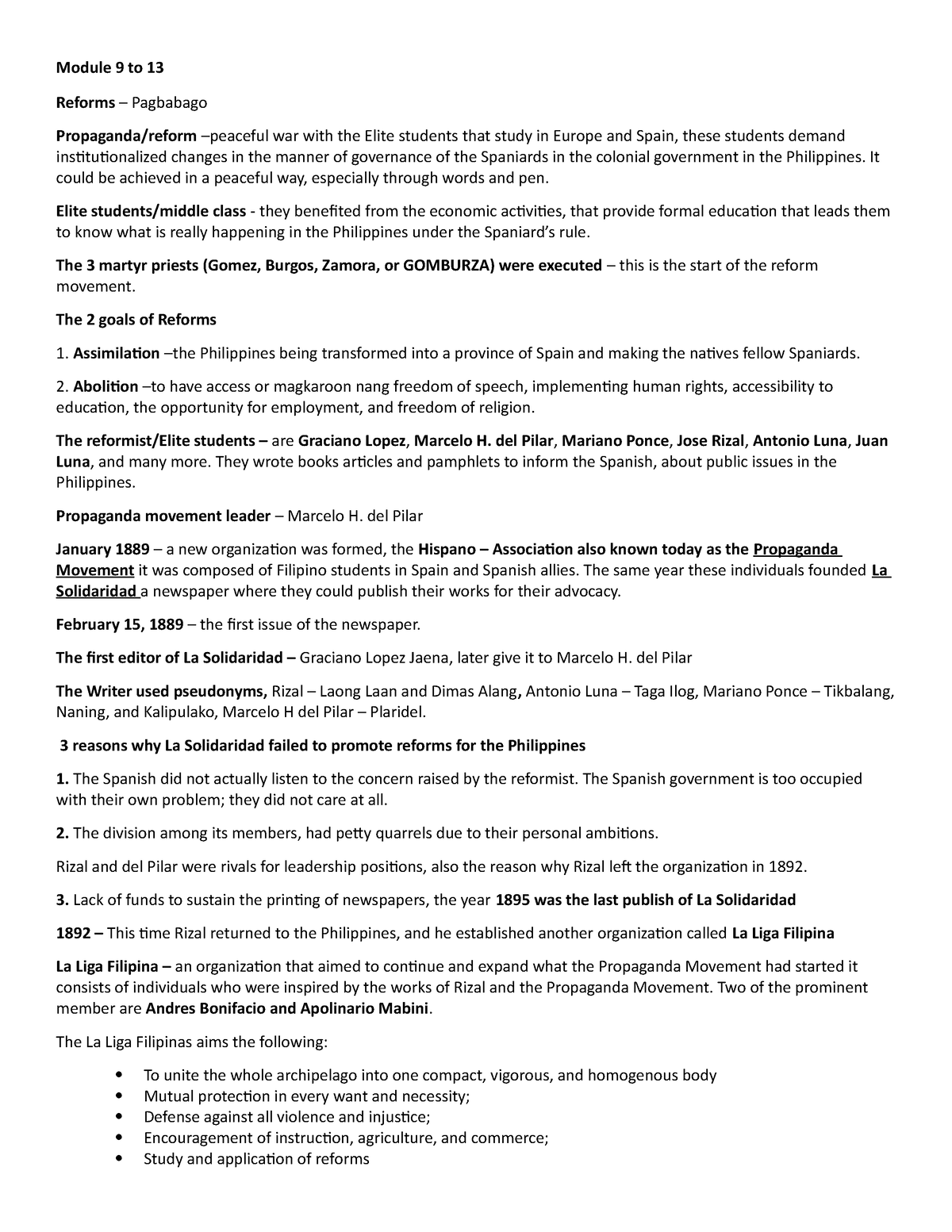This image captures a detailed list from a meeting or presentation, covering content from modules 9 to 13 with a focus on reforms. The content is organized into several key sections:

1. **Propaganda and Reform**: Discusses the intersection of propaganda efforts and reform movements, targeting elite students and the middle class.

2. **Three Martyr Priests**: Lists Gomez, Burgos, and Zamora, noting their execution.

3. **Goals of Reforms**: 
   - **First Goal**: Assimilation
   - **Second Goal**: Abolition

4. **Reformist Elite Students and Propaganda Movement Leader**: Highlights Marcelo H. Del Pilar as a significant figure in the movement.

5. **Historical Timeline**:
   - Events in January 1889.
   - The first issue of the newspaper on February 15, 1889.

6. **La Solidaridad**: 
   - Discusses three reasons for its failure to promote reforms in the Philippines.

7. **Events of 1892**: 
   - Talks about "La Lengua Filipina" and its aims, followed by detailed bullet points outlining these goals.

This list appears to be a comprehensive overview of reform-related topics discussed during a specific educational module or meeting.